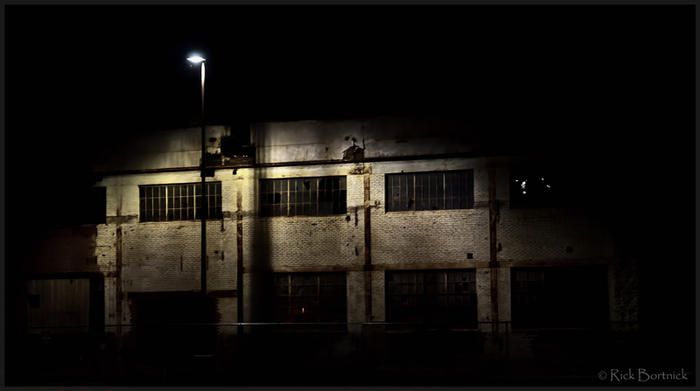This nighttime photograph depicts a two-story, possibly abandoned, building with a tall, glowing street lamp positioned to its left. The building, which resembles either an old jail or an abandoned warehouse, features broken windows and bars, adding to its dilapidated appearance. The light from the street lamp, which stands taller than the structure itself, casts a white, slightly yellowish glow on the side of the building, creating stark contrasts against the surrounding darkness. The image is composed with the building centrally framed, and the lamp slightly to the left, emphasizing the desolate and eerie atmosphere. The entire background is enveloped in black, indicating the deep night. In the bottom right corner of the image, there is a text identifying the photographer with a copyright notice: "Rick Bortnick."